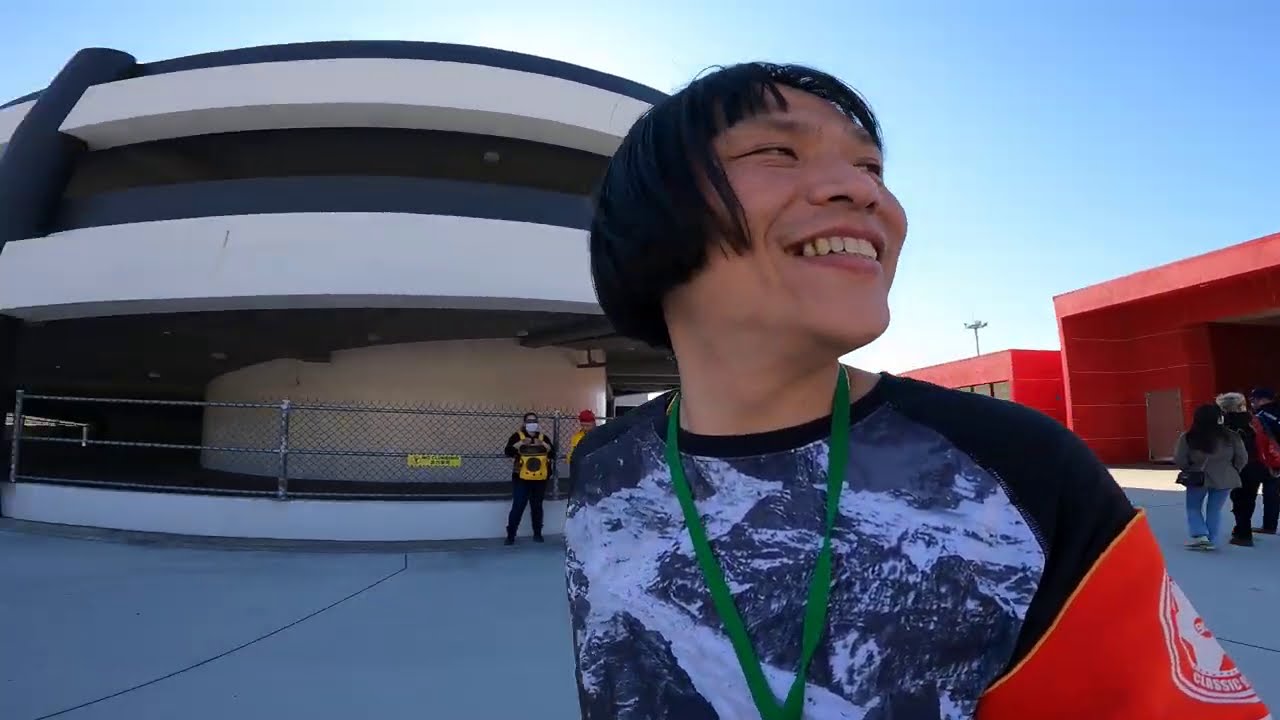In this selfie, an Asian man is seen smiling and looking over his left shoulder. He has black hair styled in a long, somewhat feminine cut. He is wearing a green lanyard around his neck and a distinct shirt featuring a white and gray camouflage pattern on the front with black sleeves. Notably, there is an orange armband on his left arm. The background reveals a square rectangular building painted mostly white with black support pillars. A man, potentially part of a security team, stands by the building wearing a white face mask, a black baseball cap, a yellow safety vest, and black pants. To the right, two square red buildings are visible. The detailed setting suggests an urban or event environment, with a fence near the white building and a few bystanders walking in the background.